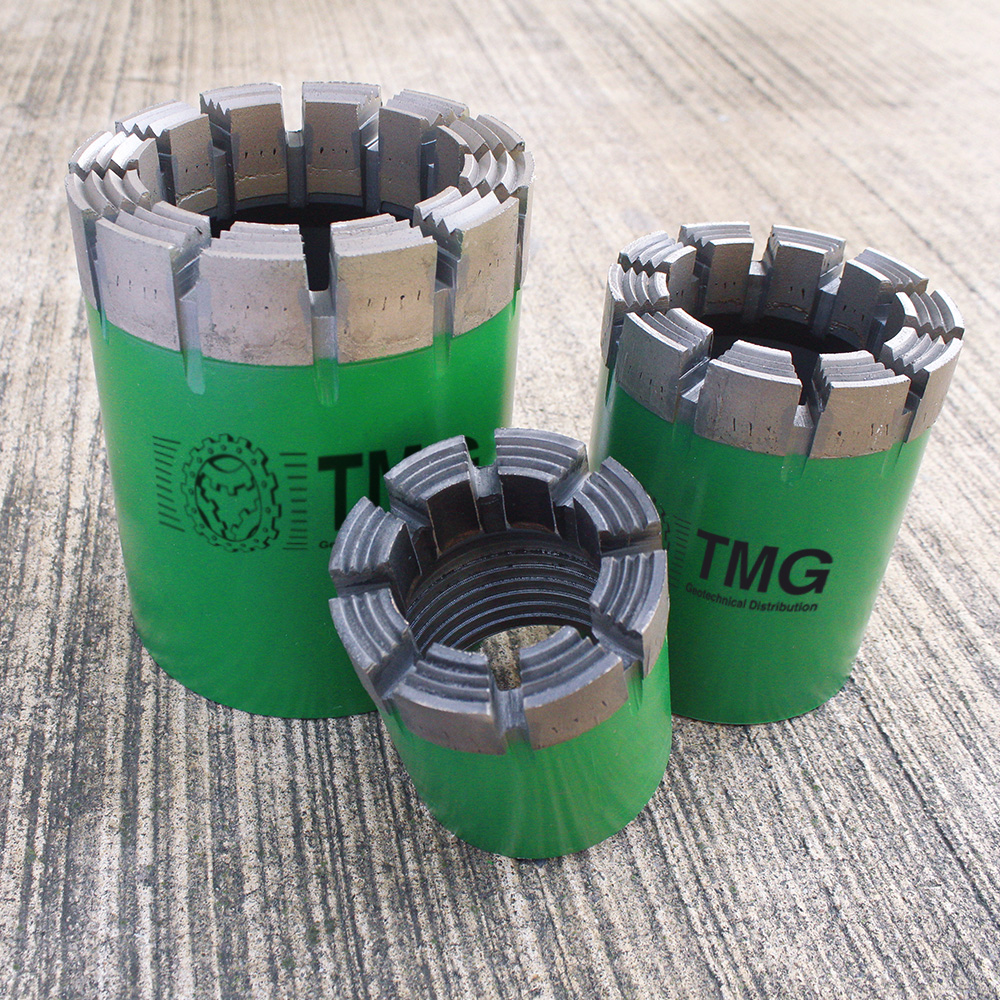The photograph features three cylindrical, green objects of varying sizes – small, medium, and large – arranged on striated beige carpeting. Each object bears the text "TMG" in capital letters, followed by "Geotechnical Distribution." The objects' design includes a prominent metal or steel top with a circular, gear-like motif, reminiscent of a rook in a chess game. The largest object also features a logo depicting a gear with slashed markings, suggestive of a globe encapsulated within. The tops have distinct teeth-like divots forming four sections, indicating they might serve as clamping devices or caps for electronic components.